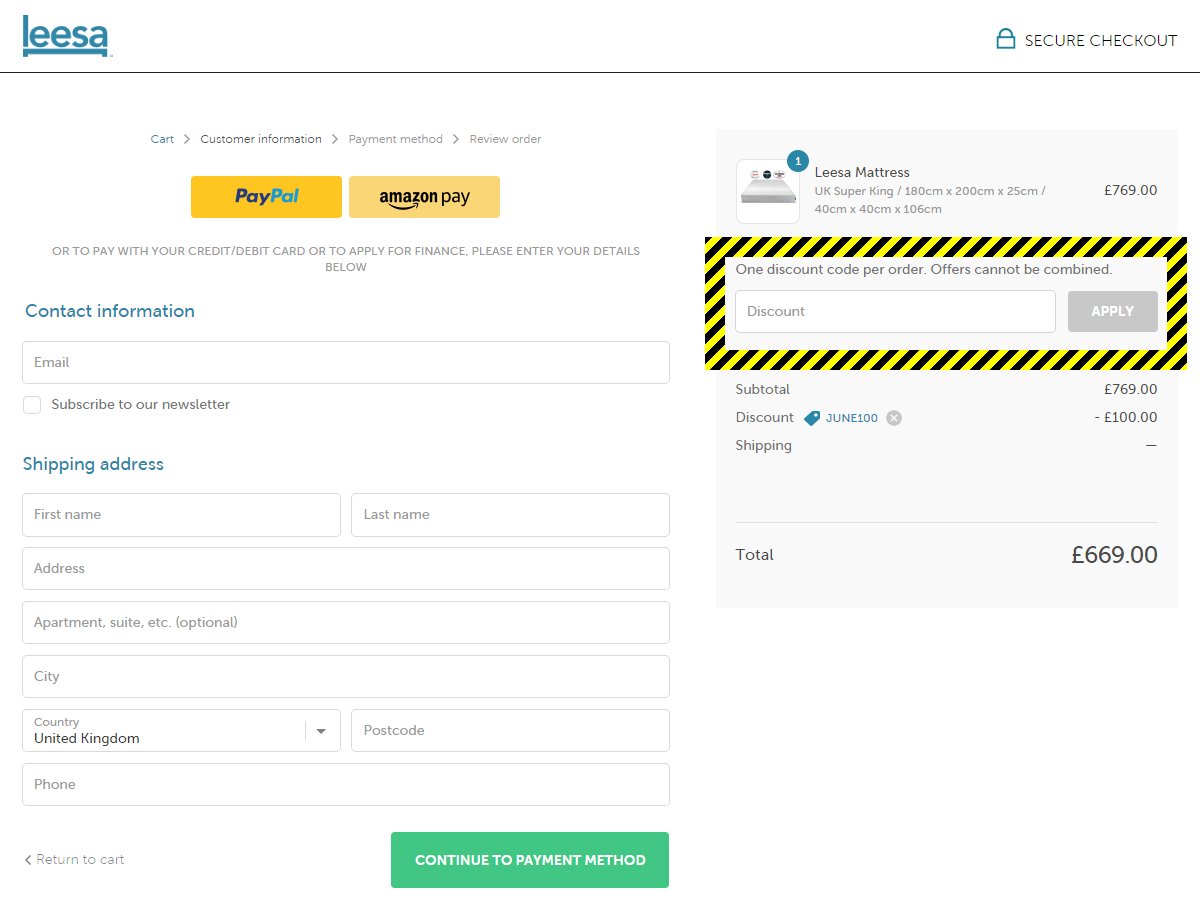A detailed screenshot from the Lisa.com checkout page shows an all-lowercase "leesa" logo in blue, located in the upper left corner above a short horizontal bracket. The right upper corner confirms it as a secure checkout page with a padlock icon. Key steps listed include: Cart, Customer Information, Payment Method, and Review Order.

Prominently displayed are two yellow buttons for PayPal and Amazon Pay. In gray font below, there's a prompt to use a credit or debit card or apply for finance by entering personal details. Fields provided for contact information include email, shipping address, first name, last name, address (with an optional field for apartment/suite), city, country (defaulted to United Kingdom), postcode, and phone number. Further down, a green button invites users to continue to the payment method.

On the right, a summary panel shows an order for a "Lisa Mattress, UK Super King (180 cm x 200 cm x 25 cm, 40 cm x 40 cm x 106 cm)" priced at £769. A field for a discount code appears below with a gray "apply" button and a caution that only one code per order is allowed. An outlined black and yellow striped rectangle emphasizes this rule. The subtotal is £769, with a discount code "JUNE100" applying a £100 reduction, bringing the total to £669. Shipping costs are marked as a dash, indicating free shipping.